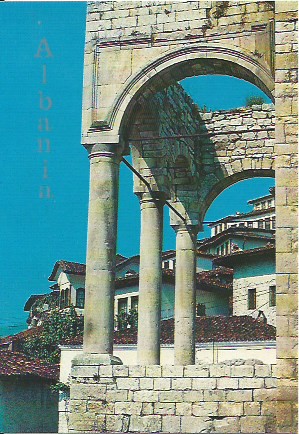The image captures an outdoor setting featuring an overarching architectural structure reminiscent of an ancient Greek Parthenon. This prominent stone and brick edifice, occupying the right two-thirds of the photo, has three grand columns rising from its base to support an arched entryway at the top. Positioned against a brilliant blue, cloudless sky, this structure also reveals a row of picturesque, single-storey white houses with characteristic stucco brown roofs, resembling those found on a Greek island. Adding to this idyllic setting, there is a hint of sparkling blue water at the base of the columns, suggesting a beachfront location. The photograph, with dimensions roughly three to four inches tall and two inches wide, appears timeless, akin to an old photograph or postcard. On the left side of the image, faint orange or grey text appears vertically, possibly spelling out "A-I-H-N-I-A" or resembling the word "Albania," enhancing the image's nostalgic and mysterious charm.